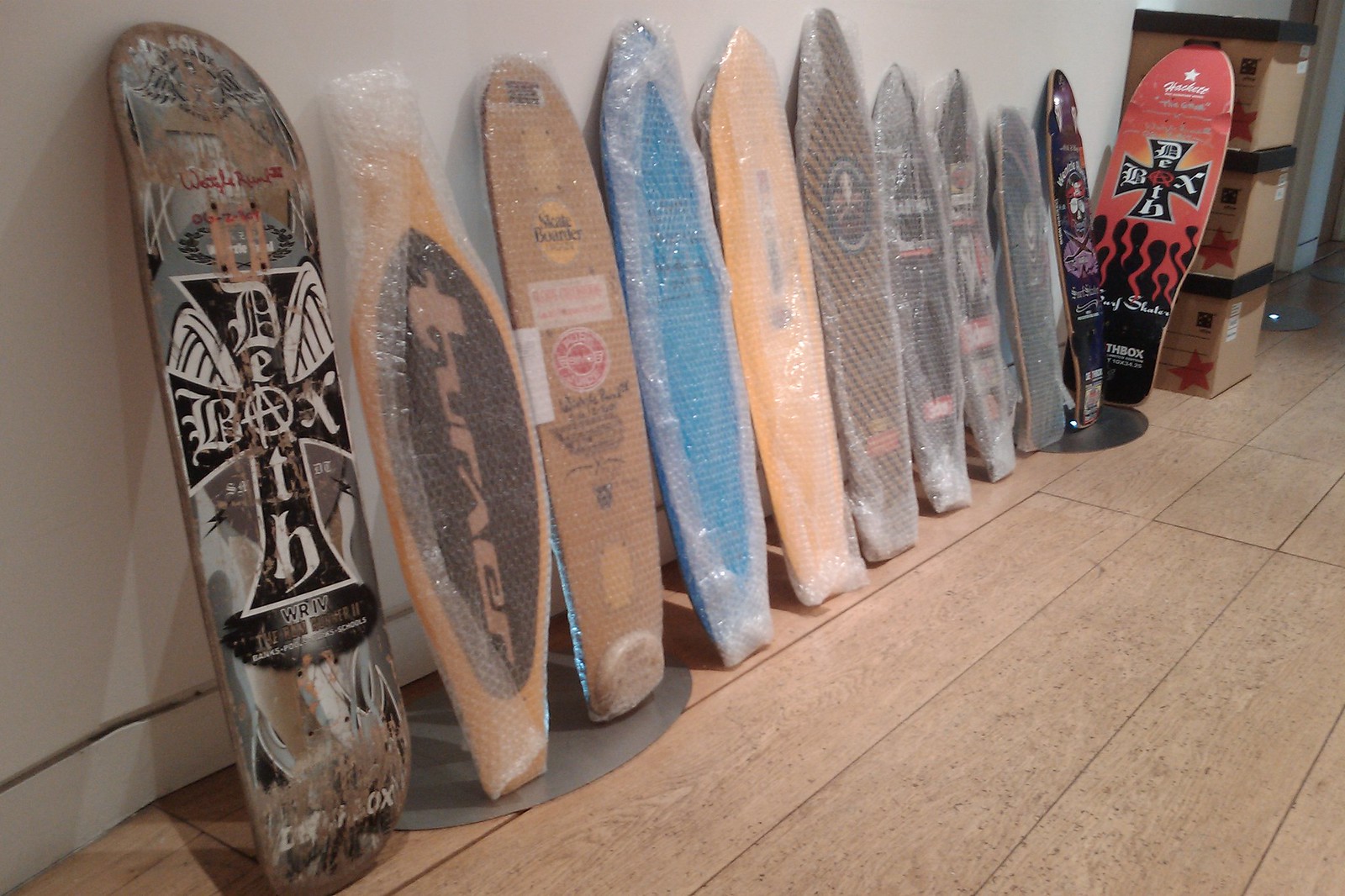The image depicts a collection of eleven skateboard decks of varying widths, thicknesses, colors, and lengths. All but one of the decks are wrapped in plastic or bubble wrap, suggesting they are new or recently delivered. The decks are leaning against a section of beige and white walls on a wide plank wooden floor, which runs diagonally from the bottom left to the upper right corner. In the upper right corner, there are three cardboard boxes with darker lids stacked atop each other, against which the only unwrapped, seemingly used red skateboard deck leans. The remaining ten decks form a neat lineup against the wall, with the first deck on the far left featuring a cross and possibly the words "Death Ray" or "Death Box." Next to it, a light brown deck with black lettering spells out "Tour," followed by a brown board, a blue board, a very light-colored board, and progressively darker boards. The overall setting appears to be the back room of a skateboard shop, suggesting an inventory check or a recent arrival of new products.